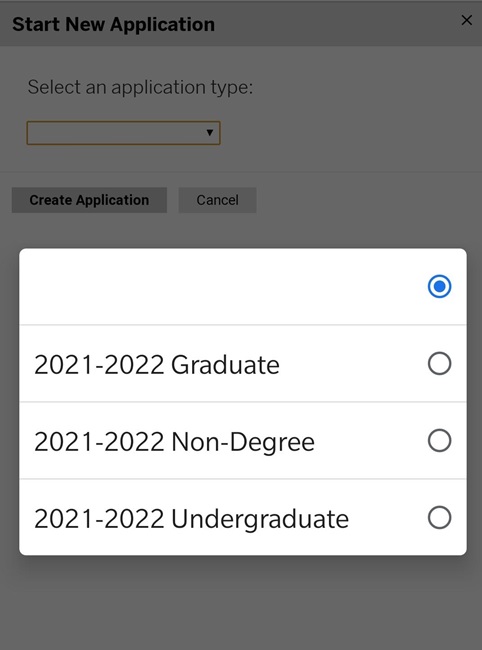The image showcases an online application process interface. The background is predominantly white, with text positioned in the top left corner that reads “Start New Application” in black font. Directly below this text is a dropdown menu labeled “Select an application type,” which is currently highlighted in yellow, indicating that it has been clicked. Beneath the dropdown are two buttons: "Create Application" on the left side and "Cancel" on the right side.

At the bottom of the image, there is a popup menu extending from the selected dropdown, presenting four options. The first option is empty but has a blue check dot indicating it is selected. The subsequent options are labeled as follows: “2021 to 2022 Graduate,” “2021 to 2022 Non-Degree,” and “2021 to 2022 Undergraduate,” none of which are highlighted or selected.